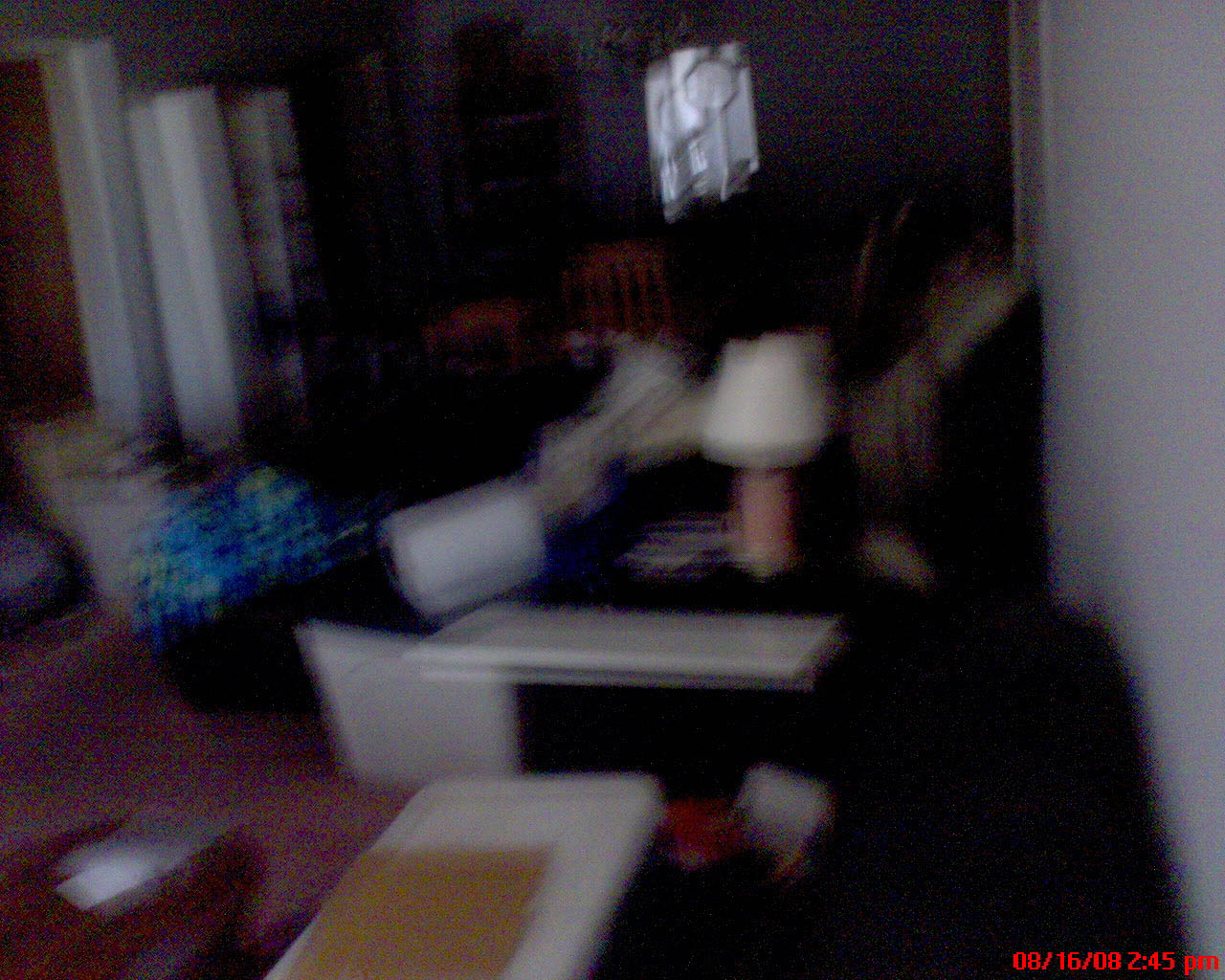This image depicts a living room captured in a very blurry photograph, likely due to the camera being moved too swiftly at the time of the shot. The room appears dimly lit, accentuating the blur caused by the motion. The timestamp in red text on the bottom right corner indicates it was taken on August 16, 2008, at 2:45 p.m., suggestive of the era's less advanced camera technology. The living space features various pieces of furniture - a lamp, a couch, and a dining table surrounded by wooden dining chairs are discernible. Taller furniture items, possibly bookcases, are also visible, and there is a doorway on the left leading to another room. The overall ambiance reflects a typical, lived-in living room from that period.